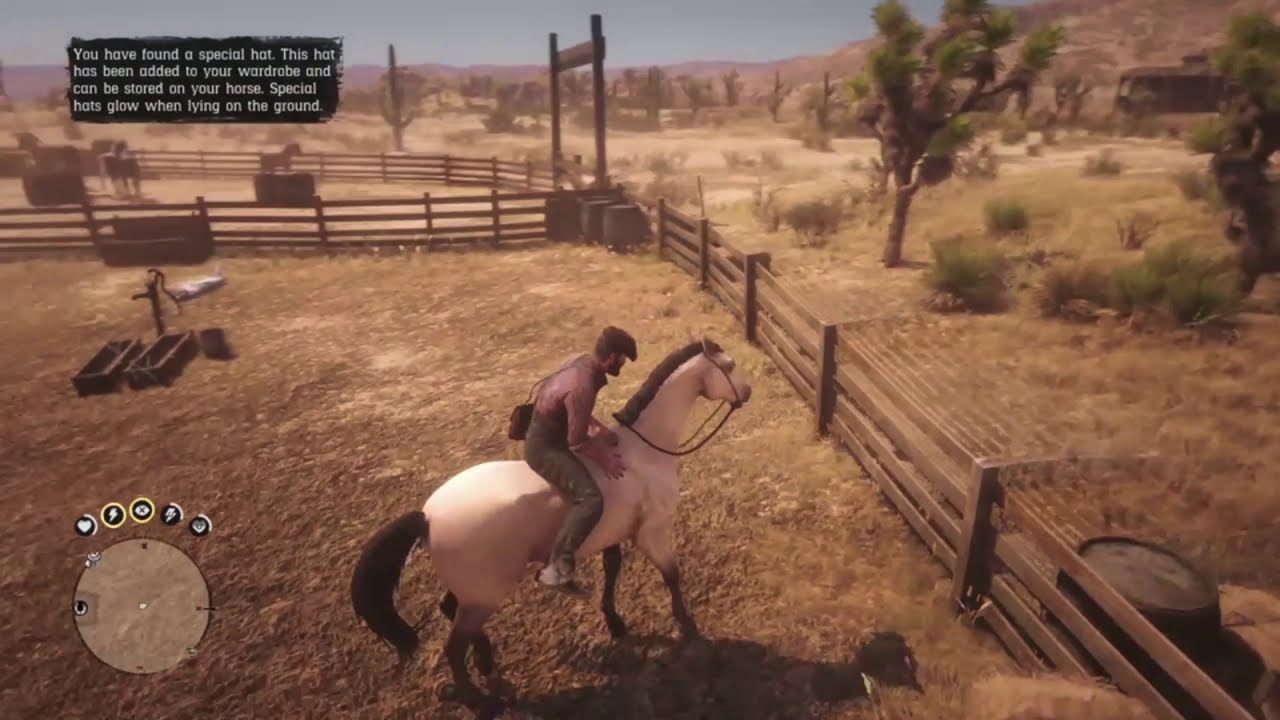In this detailed screenshot from a video game, we see a man riding bareback on a striking white horse with a black mane and tail. The man, attired in a purple shirt, gray pants, boots, and a flat-tam hat, appears to be exploring a desert-like setting. This area features cacti, small shrubs, and brown, dirt-filled ground, encapsulated within a wooden fence that forms a corral. In the upper left corner of the screen, a black text box with white font reads: "You have found a special hat. This hat has been added to your wardrobe and can be stored on your horse. Special hats glow when lying on the ground." The bottom left corner displays a mini-map with various icons. In the distance, a mountain range and scattered buildings can be discerned, enhancing the realistic and immersive nature of the game's environment.